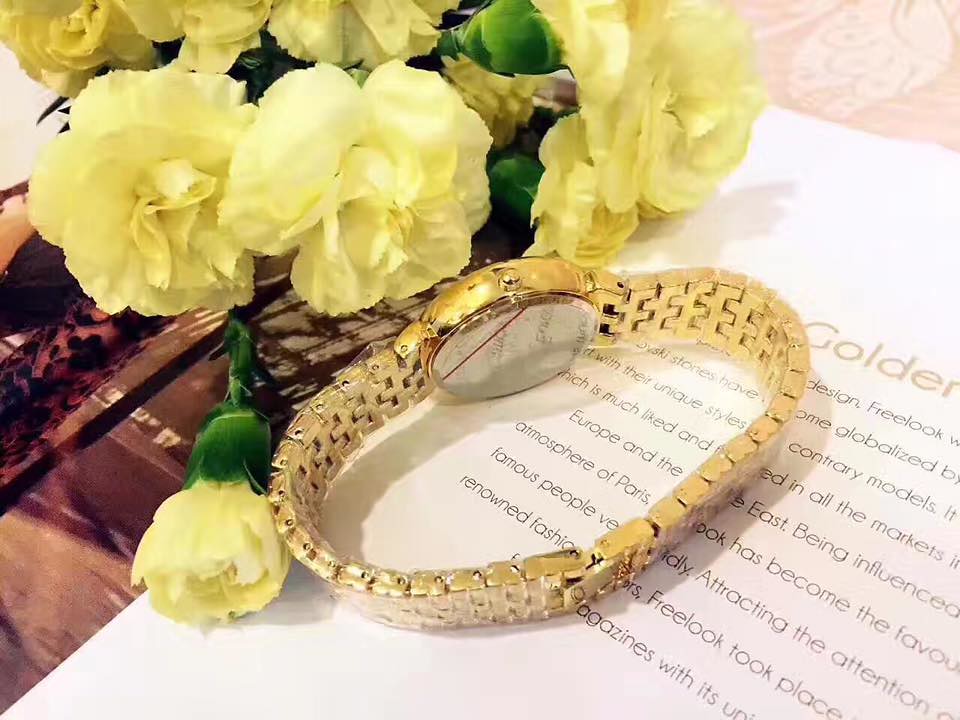In this photograph, various items are meticulously arranged on a table with a pink-patterned tablecloth. Prominently, there is a golden chain-link watch placed over a white sheet of paper. A noticeable portion of the paper's text reads, "Freelook stones have globalized their unique styles, contrary models, which is much liked and in all the markets. Europe and the East being influenced atmosphere of Paris has become the favor. Famous people attracting the attention. Renowned fashion, Freelook took place with its," though parts are obscured by the watch and the image frame. Adjacent to the watch, on the upper left stretching to the middle, are pretty light yellow flowers, with one not yet fully bloomed, set delicately on the table. The combined elements of the golden watch, yellow flowers, and the partially visible textual paper create a harmonious and elegant scene.